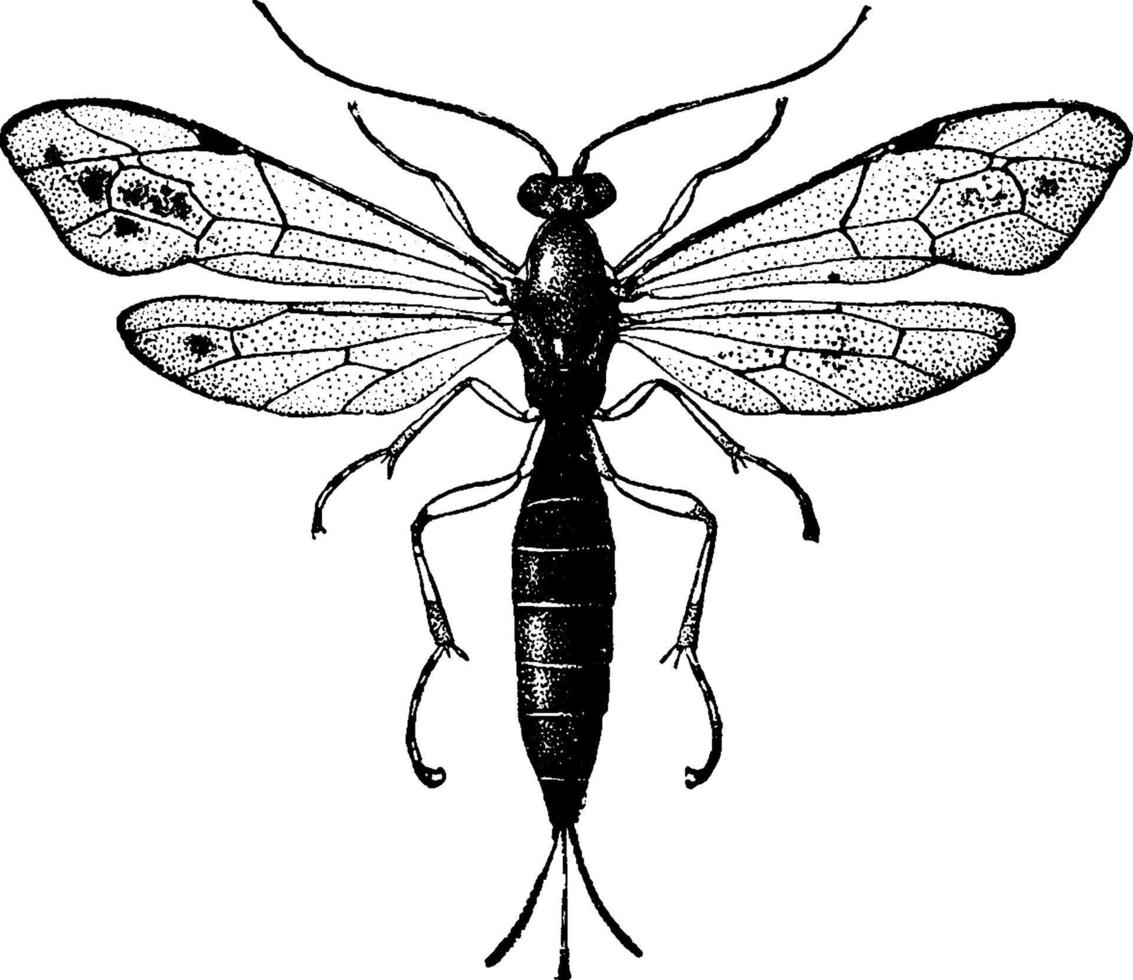This image is a highly detailed black and white illustration of a flying insect, likely resembling a moth. The insect is viewed from above, highlighting its distinct anatomical features against a white background. It possesses a long, oval-shaped head with two lengthy, thick antennae extending sideways. The body, entirely black, comprises a long, skinny torso and an extended abdomen from which three thin, tail-like extensions emerge.

The insect's wings are a defining feature, consisting of two sets on each side. The upper wings are larger, while the lower wings are smaller. Although the wings are primarily translucent, they contain black dots and thin black lines, particularly along the edges, providing a detailed contrast against their transparent nature.

The insect has six legs in total: two at the front, two in the middle, and two towards the rear of the body. This intricate rendition of the insect captures the essence of its form with meticulous attention to detail, illustrating the delicate balance between its black body and the white expanse surrounding it.